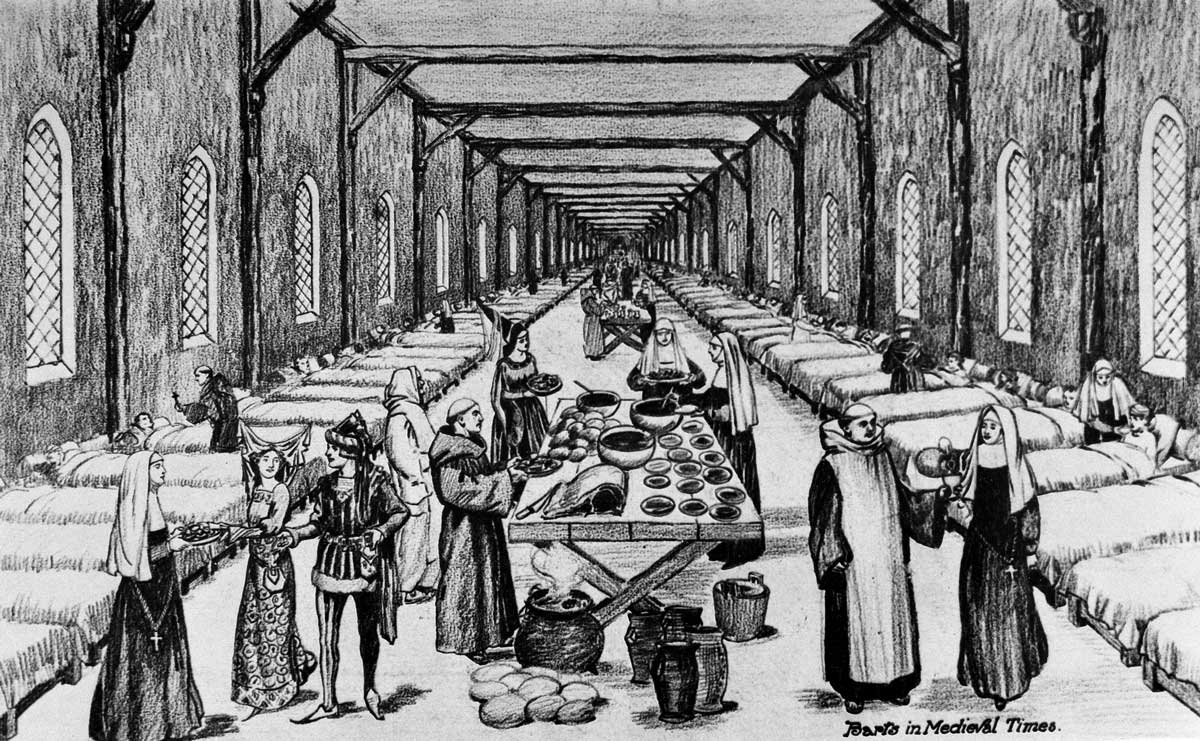The image is a meticulously detailed black and white drawing of a scene in a medieval hospital, identified as "Barts in Medieval Times" in the bottom right-hand corner. The center of the drawing features a large table laden with food, including large bowls, plates, and steaming pots, surrounded by nuns in habits, monks, and other figures, including a jester in a court jester outfit and women in elaborate dresses. Surrounding the central table are rows of beds along both the left and right sides of the image, each bed occupied by patients being attended to by the nuns. The setting bears an air of brightness and clarity, with arched windows providing ample natural light, suggesting a church-like ambiance. The architectural details such as wooden beams add to the medieval atmosphere, while the crowded arrangement of beds emphasizes the crude nature of the hospital. The scene combines the hustle of a medieval feast with the solemnity of a hospital ward, capturing a vivid snapshot of life in medieval times.